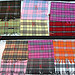This image showcases a collection of twelve small, intricate checkered patterns arranged in an organized fashion. These designs are displayed both on the wall and on the floor. In the top left, there is a black and gray checkered pattern with intersecting lines. Adjacent to it on the right, a checkered motif combines pink and blue hues. Next, another pink and blue checkered design follows. Continuing right, a dark pink and light blue crisscross display adds variation. Just below, two carpets feature green and yellow checkered patterns. To the right of these, a dark pink, almost magenta, and blue checkered pattern stands out. Further down, a yellow and blue checkered design catches the eye. Another pink and blue pattern can be seen in the middle. Adjacent to it, a checkered carpet with orange and green colors stands out with its vibrant hues. Present is another pink and blue design, and a dark gray and light gray checkered pattern with red accents follows. The final piece on the bottom right includes a stark white and black checkered pattern. Together, these twelve checkered images create a visually captivating array of colors and patterns.